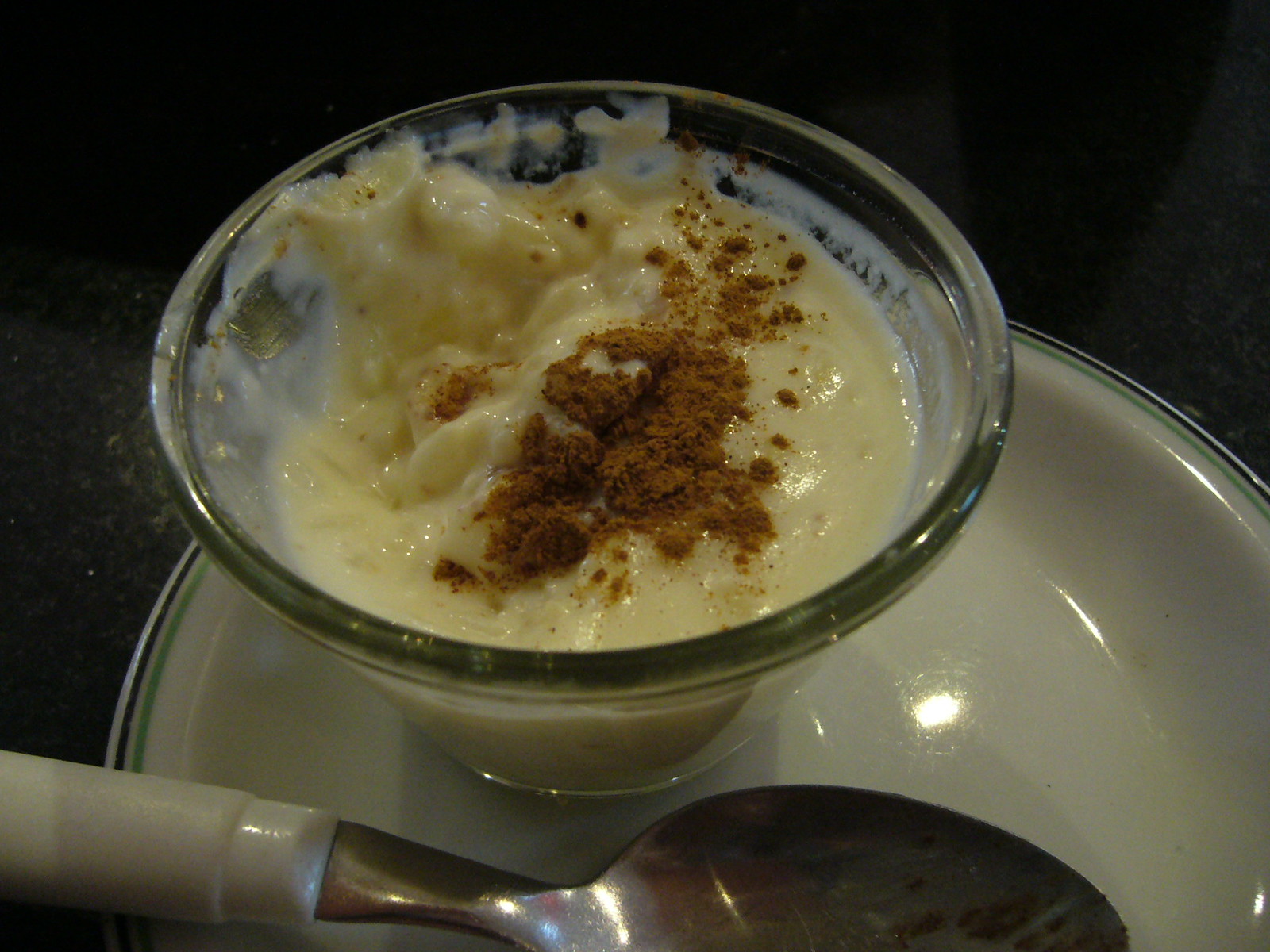This image is a very detailed close-up photograph of a homemade dessert. The dessert, which is likely vanilla or rice pudding, is presented in a small glass dish that is set on a white plate. The plate features a green circle and a black line trim around its perimeter. There is a generous sprinkling of cinnamon on top of the pudding, giving it a rich, inviting look. The dish is accompanied by a clean silver spoon with a white plastic handle positioned next to it on the plate. The pudding appears to have had a few bites taken out of it, with some slight smearing visible on the spoon. The background is dark, possibly a black marble countertop, suggesting subdued lighting conditions. The close-up nature of the photo highlights the pudding's creamy texture and tiny bubbles, emphasizing the homemade quality of the dessert.